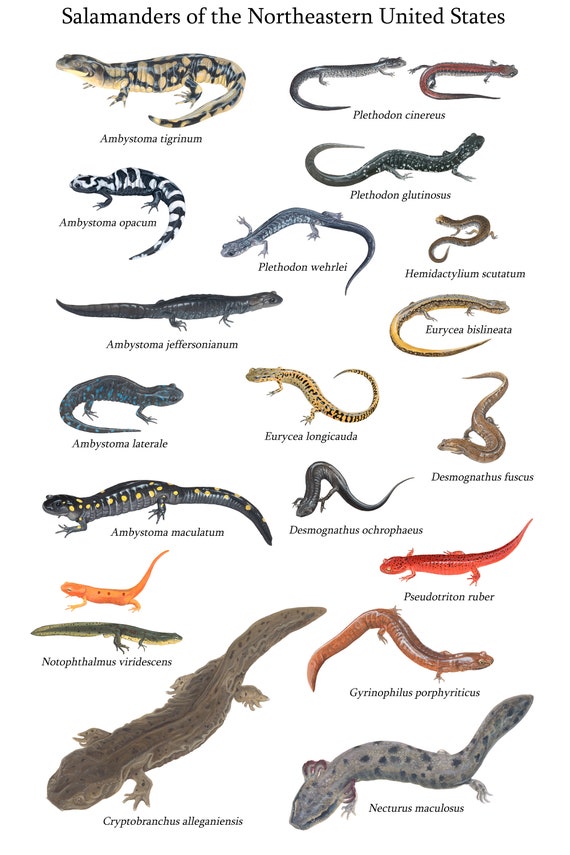The image is a detailed educational chart titled "Salamanders of the Northeastern United States," featuring photorealistic pictures of approximately 13 different types of salamanders. Each salamander is distinctly colored, showcasing a variety of hues including bright oranges, grays, browns, blues, greens, and multicolored patterns. Some notable examples include a yellow salamander with black spots, a white one with black spots, a brown bluish one, a black and blue one, and a completely black one with yellow spots. Other salamanders are entirely orange, green and blue, all brown, bright red, and completely black. These salamanders not only vary in color but also in size and shape, with some resembling worms with elongated bodies and others exhibiting differing numbers of claws and tail sizes. The names of each species, which are quite long, are displayed beneath their respective images, making this chart an excellent resource for anyone wanting to learn about the specific breeds and characteristics of salamanders from this region. It’s ideal for science classes or enthusiasts looking to identify and understand the diversity of salamanders in the Northeastern United States.